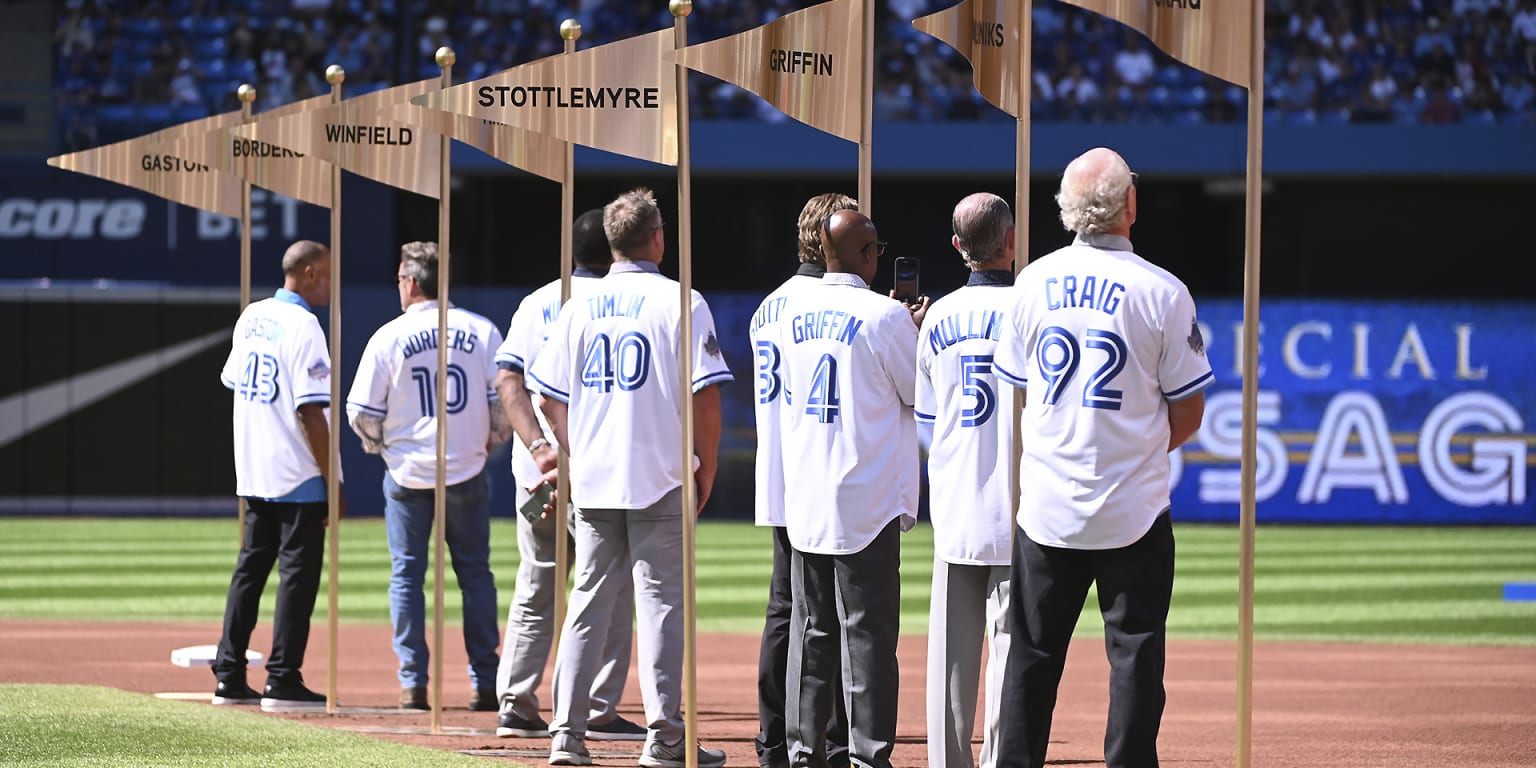The photograph depicts a professional baseball field during a special ceremony featuring a group of eight retired players, likely from the Toronto Blue Jays, based on the context. These older gentlemen are all standing in the infield, facing the stands, which are filled with spectators too distant to distinguish clearly. Each player wears their respective jersey, displaying their number and last name on the back. Standing next to each player is a flagpole bearing a brownish or black flag with their surname on it. Notable players such as Dave Winfield, wearing jersey number 10, and Craig Griffin, wearing jersey number 4, can be identified among the group. The green field, accented with areas of sand, further confirms the setting as a baseball stadium. The players' solemn posture, with most having their arms in front of them, suggests this is part of an on-field ceremony, possibly honoring their contributions to the sport or commemorating their entry into a Hall of Fame.